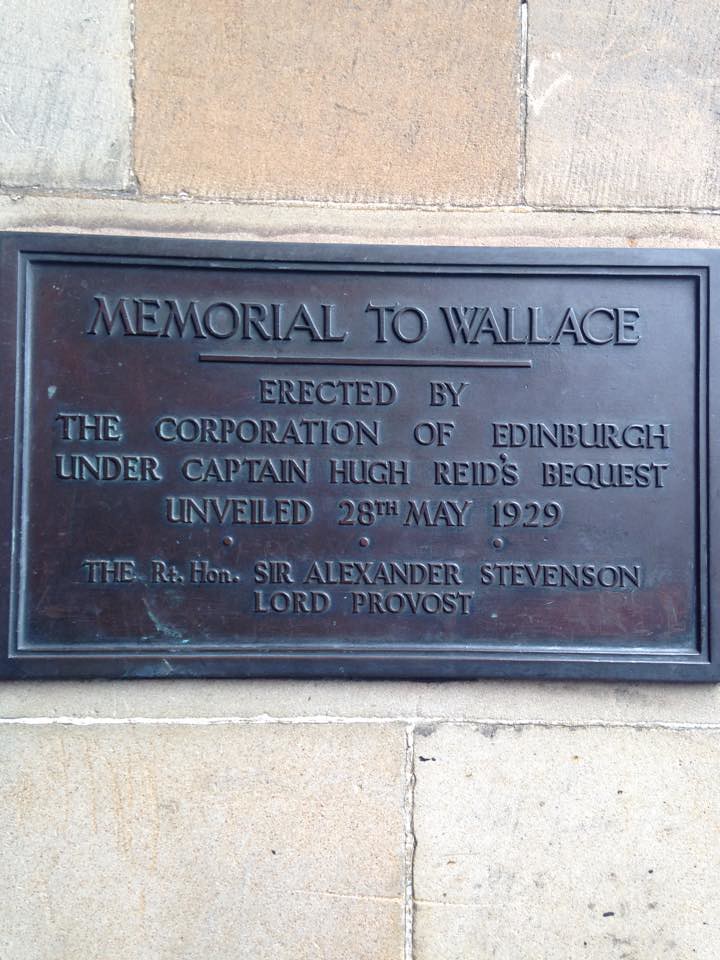The image depicts a bronze plaque embedded on the side of a stone wall. The wall appears to be part of a building, constructed from large, grey stone slabs with a hint of reddish tint at the top, and distinct brick outlines. The plaque, dark and aged, features embossed text and an embossed frame, both standing out in a 3D effect against the bronze background. The inscription on the plaque reads: "Memorial to Wallace," underlined by a horizontal raised line. Below this, the text continues: "Erected by the Corporation of Edinburgh under Captain Hugh Reid's Bequest, unveiled 28th May 1929." Further down, it states "The Rt. Hon. Sir Alexander Stevenson, Lord Provost," signifying the formal dedication by the honored person. The photograph focuses primarily on this commemorative plaque, leaving the rest of the building outside the frame.